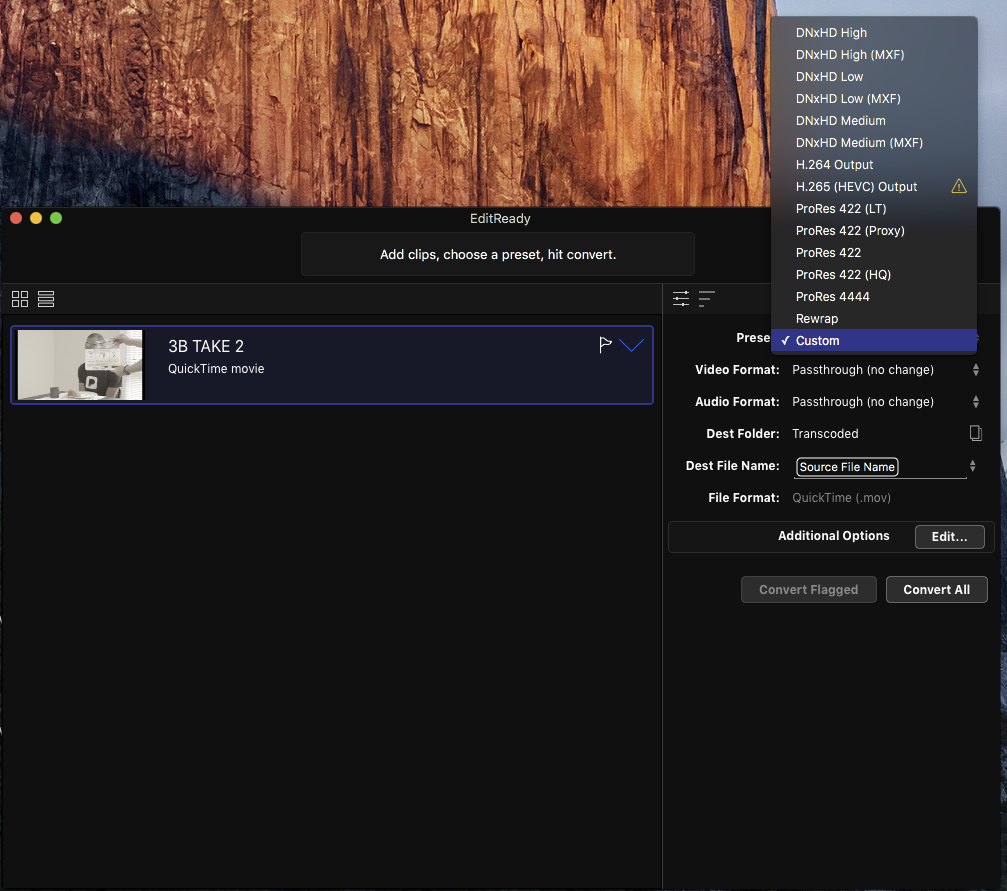The image depicts the interface of a program, likely named "EditReady." In the top left corner of the window, there are three round buttons: red, yellow, and green. The interface header includes buttons labeled "Add Clips," "Choose a Preset," and "Convert." 

On the bottom section of the interface, there is a preview of a QuickTime video file titled "3B Take 2," which is enclosed in a blue box with a blue checkmark. On the right side, there are multiple settings options available, including preset video format, audio format, destination folder, file name, file format, additional edit options, and buttons for "Convert Flagged" and "Convert All."

Currently displayed is a list of different video format presets, such as DNxHD High, DNxHD Low, DNxHD Medium, H.264, ProRes 422, and Rewrap. 

In the background, the desktop wallpaper shows a panoramic view of a mountainous region with sunlight illuminating the brown terrain, giving it a picturesque appearance.